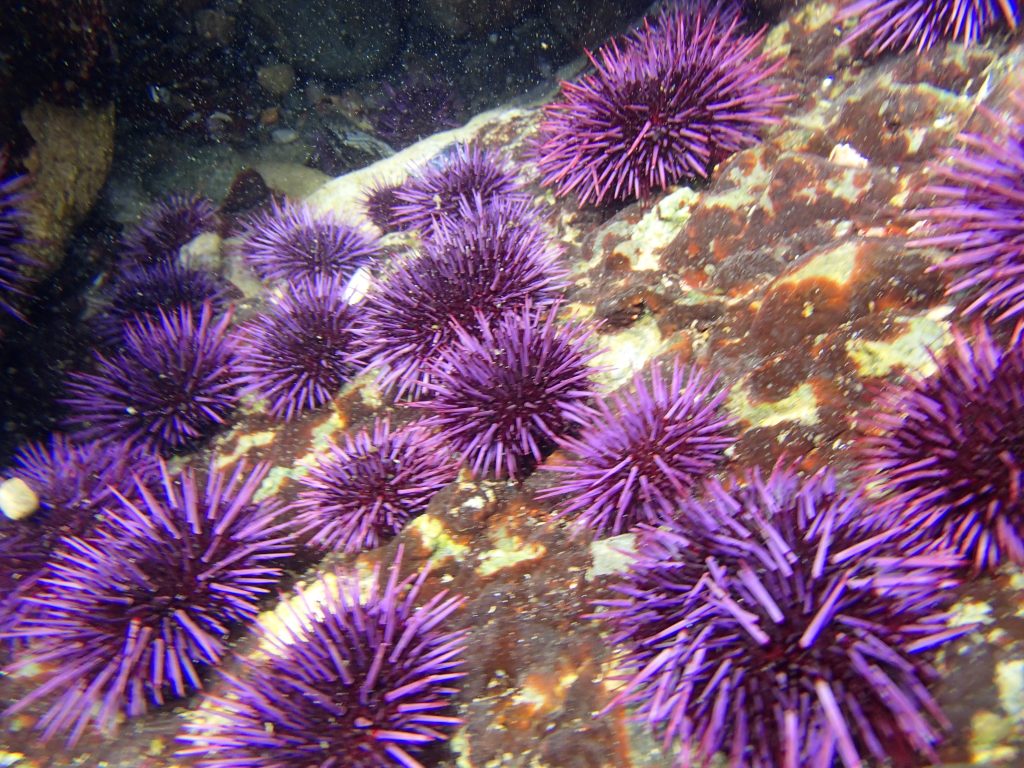This underwater photograph showcases a richly detailed view of a seabed teeming with marine life. The focal point is a cluster of sea urchins, vividly colored in purple with pink-tipped spines, set against a beige seabed mottled with splotches of brown and red. The water is filled with particulate matter, creating a grainy texture thanks to specks of brown and white floating throughout. Behind the urchins, a colorful array of rocks in shades of brown, red, gray, and beige adds depth to the scene. The well-lit foreground, likely illuminated by the photographer, contrasts sharply with the darker background where more urchins are visible. There's a suggestion of black moss interspersed with the sea urchins, further enriching the intricate marine tableau. A potential reflection hints at the possibility that this image might be taken inside a tank, adding a layer of intrigue to the natural beauty on display.